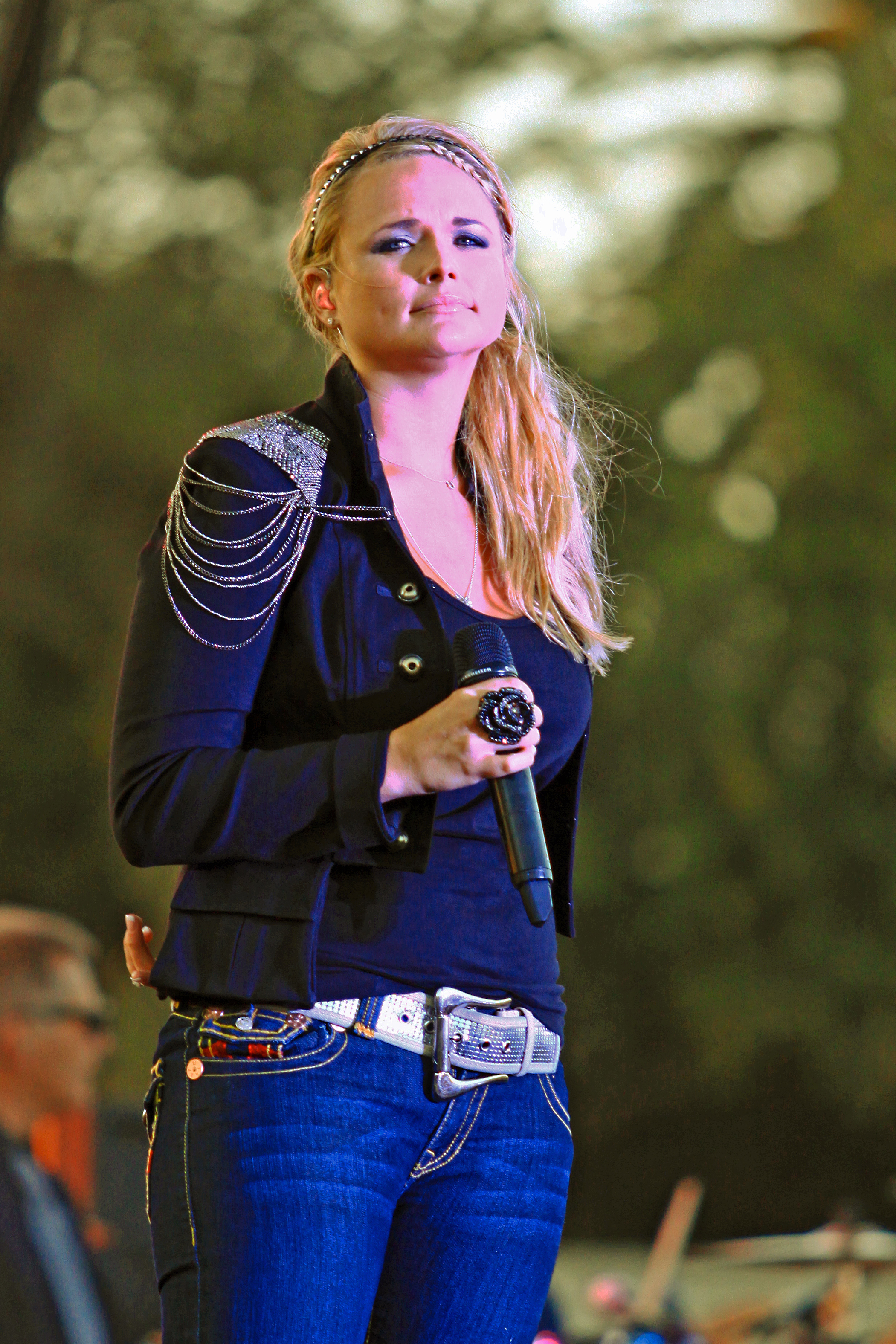The image features a young Caucasian woman, likely in her 20s or 30s, standing from mid-thigh up to the top of her head. Her body is angled slightly towards the five o'clock position, but her head is turned to face the viewer. She has long blonde hair cascading down to her chest, with a thin headband and a single braid in the front. She's adorned with purple eyeshadow and pink lipstick.

She's dressed in a stylish blue outfit consisting of a blue tank top underneath a blue blazer decorated with cascading shoulder pads. Her ensemble is completed with blue jeans and a white belt with a metallic buckle. Her right hand is bent at a 90-degree angle in front of her chest, holding a microphone, which is black with a dark green and dark blue top. On her middle finger, she wears a sparkling jeweled flower ring.

In the background, a blurry green tree adds a touch of nature to the scene. The woman appears to be a country singer, with details suggesting she might be Miranda Lambert.